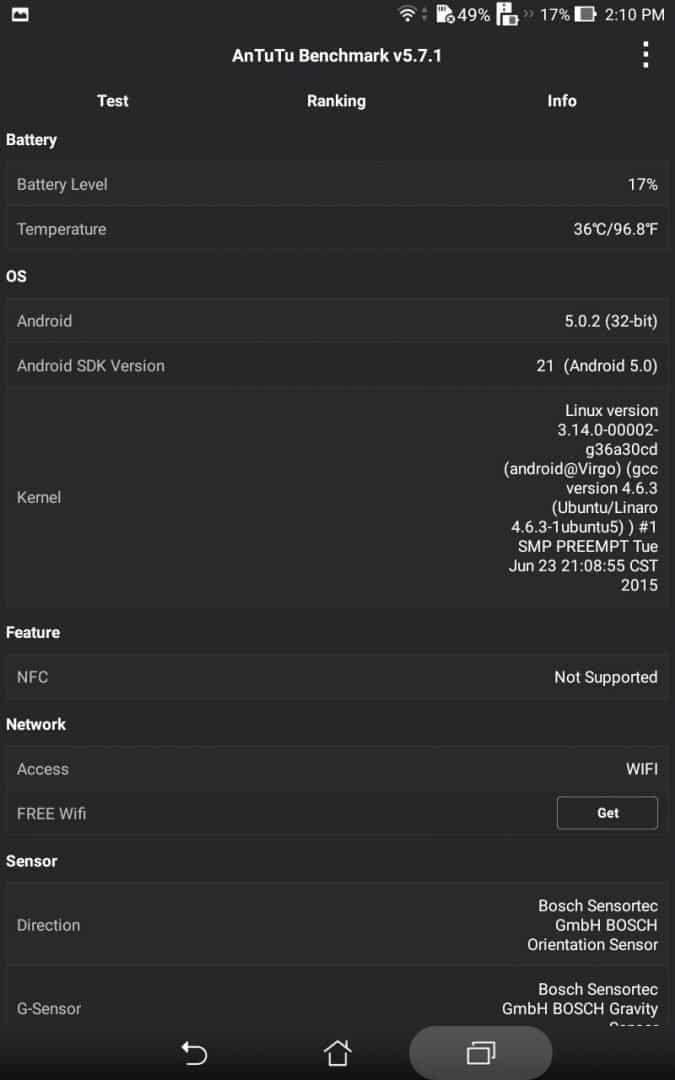This image is a screenshot taken from a mobile device or tablet displaying detailed system information. Along the top of the screen are icons indicating the Wi-Fi connection, battery status (17%), and the current time. The bottom of the screen features three navigational buttons: a back arrow, a home button, and a recent apps button. The screenshot has a black background with predominantly white text and is densely packed with information.

The main content is titled "AN22 Benchmark Version 5.7.1" and is presented in a table format with three columns. These columns provide ranking information on various software and hardware elements of the device. Key details include the battery level (17%) and temperature (36°C), the operating system (Android Version 5.0.2 32-bit), and various feature sensors and network information. The layout is methodical, organizing critical data points for easy readability and analysis.